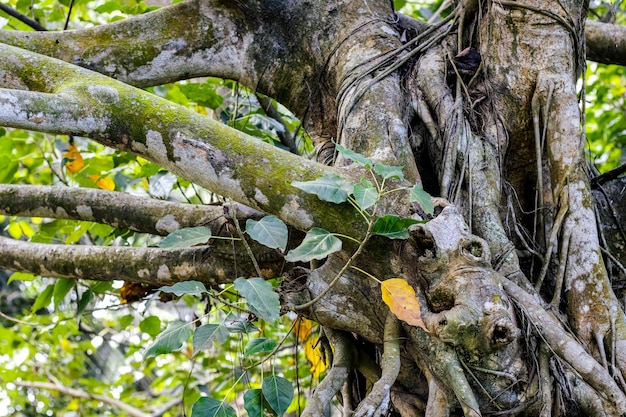The image showcases a close-up of a thick tree trunk from its upper portion where the branches start to split off. Most of the upper trunk and limbs are covered in lush green moss, creating a rich, textured surface. A single yellow leaf is visible amidst the green foliage, highlighting the transition of seasons. The main section where the trunk branches out features deep recesses that cast dramatic shadows, adding depth to the composition. This main trunk section has a small offshoot with green leaves, positioned over the base trunk just before a larger moss-covered limb diverges toward the left.

The background, blurred to emphasize the foreground, suggests a bright, sunny day with an array of leaves from other trees, reinforcing the natural setting. The trees dominate the image, with detailed textures of rough bark, foliage, and moss. Thin vines intertwine with the green leaves, and sporadic holes and small roots add to the complexity of the scene. Overall, the image is a vivid depiction of nature's intricate beauty and the tree's robust structure.